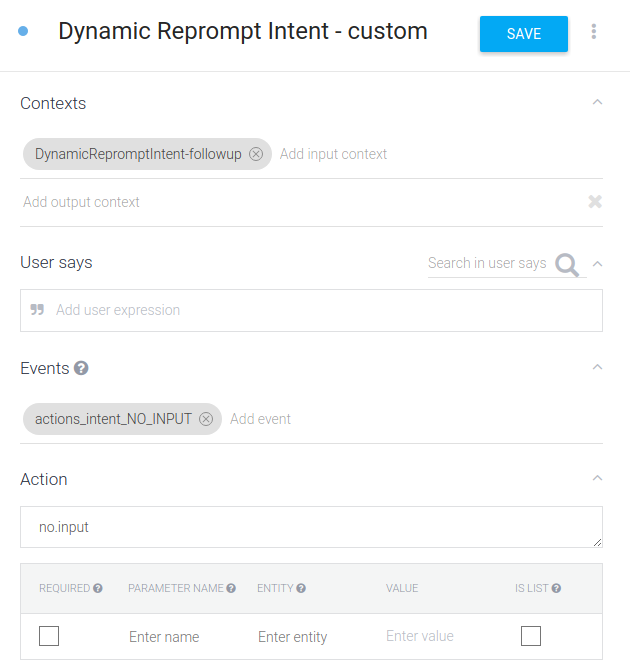This image appears to be a screenshot of a "Create Report" interface in a software application focused on configuring a dynamic reprompt intent. At the top of the page, there is a blue dot accompanied by the text "Dynamic Reprompt Intent - Custom." Next to this, a blue button with white lettering reads "Save," with three vertically aligned dots beside it, likely indicating a dropdown menu for further options.

Below this section, there is a label for "Contexts," which appears to be greyed out, indicating it isn't currently editable or accessible. The next line displays "Dynamic Reprompt Intent Follow-up" with an 'X' to the right, highlighted in grey. Following this, the interface offers options to add "Input Context" and "Output Context" respectively.

Moving further down, there is an input field labeled "User Says" in quotation marks, which seems to be relevant for entering search queries or commands. The phrase "Search in 'User Says'" is suggested within this field. Directly below, there is a section labeled "Events" followed by a question mark and the text "Actions Intent No Input." 

Additionally, the interface includes options for "Action No Input" and other menu items beneath them. In the subsequent section, there are fields and checkboxes for specifying parameters: "Required Parameter Name," "Entity," "Value," and a selection indicator for "Is List." Two smaller boxes follow this, allowing the user to enter values for "Name," "Entity," and "Value," with the provision to check the relevant option.